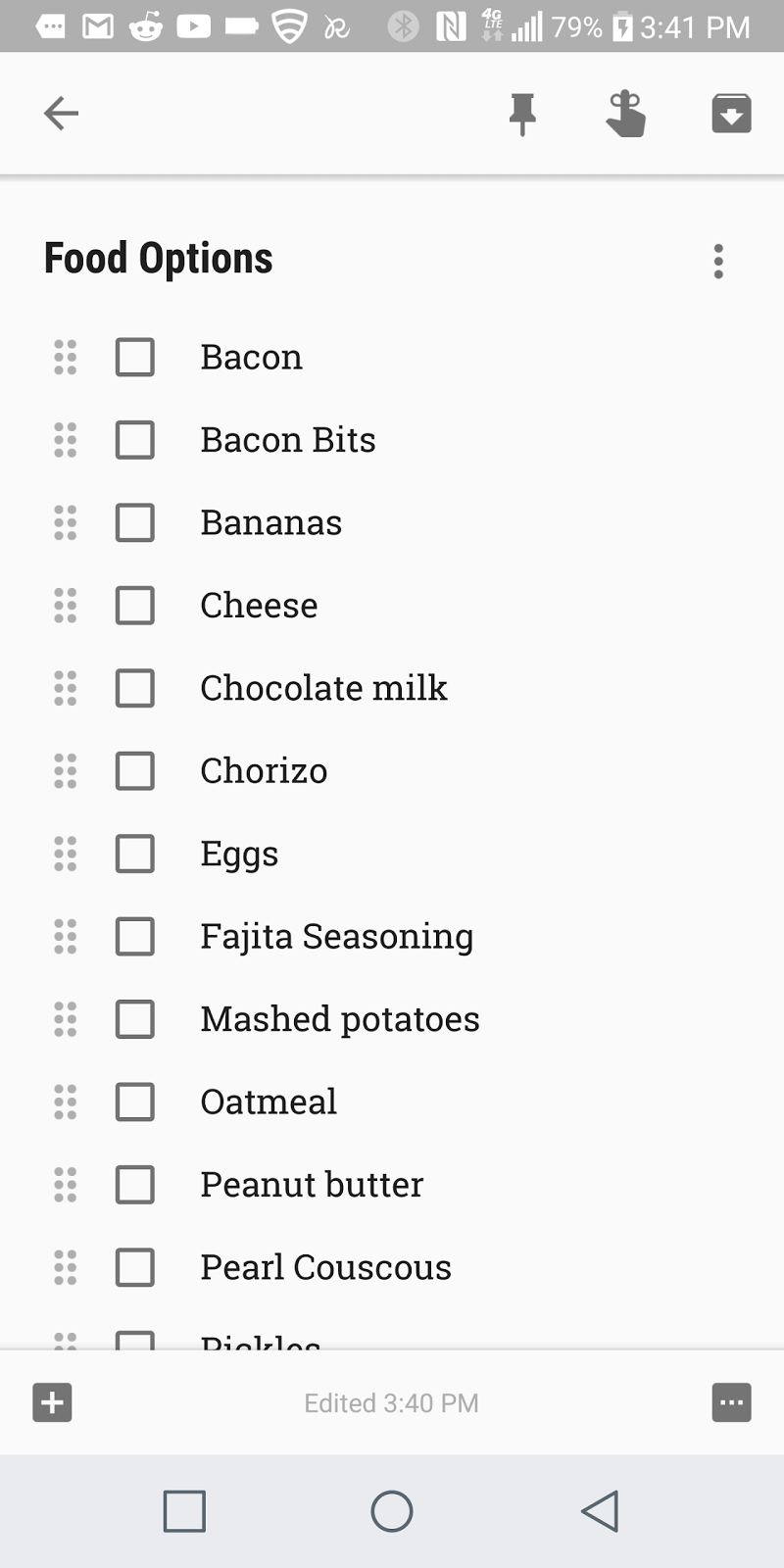The image is a screen capture of a smartphone taken at 3:41 PM, displaying a battery charge level of 79%. At the top of the screen, numerous notification icons are visible. The focal point of the image is an app featuring a list of food items under the title "Food Options." An arrow icon is also present, indicating the option to navigate back to a previous screen.

The list of food items is as follows:
1. Bacon (with a checkbox next to it)
2. Bacon bits
3. Bananas
4. Cheese
5. Chocolate milk
6. Chorizo
7. Eggs
8. Fajita seasoning
9. Mashed potatoes
10. Oatmeal
11. Peanut butter
12. Pearl couscous
13. Pickles

The items listed do not seem to be related to a specific recipe or meal type, suggesting that the app may be for ordering diverse groceries for delivery rather than ingredients for a particular dish, such as a salad.